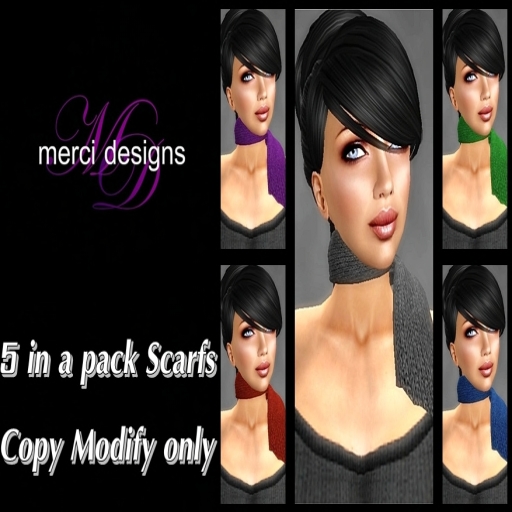The image serves as an advertisement for a five-pack of scarves by Mercy Designs. The left side of the image features the brand name "Mercy Designs" in white font, accompanied by the logo "MD" in purple cursive, with the "M" positioned higher than the "D." Below this, the text reads "Five in a Pack Scarves, Copy, Modify Only." The main focus is on a series of five images displaying the same woman modeled in a digital format, likely from a video game like The Sims, showcasing the scarves in different colors: purple, red, gray, green, and blue.

The woman, portrayed from her chest up, has stylishly done black hair and bangs that swoop across her face, covering one eye in a fashionable manner. Her hair appears to be tied up, emphasizing her facial features, which include smoky eyes, pink and black eyeshadow, big lips painted pink, and very blue eyes. She wears a gray and black shirt, and in each image, the scarf is tied high up on her neck.

The layout includes a central, vertically stretched image of the woman, flanked on all four sides by smaller images displaying each scarf color variation.